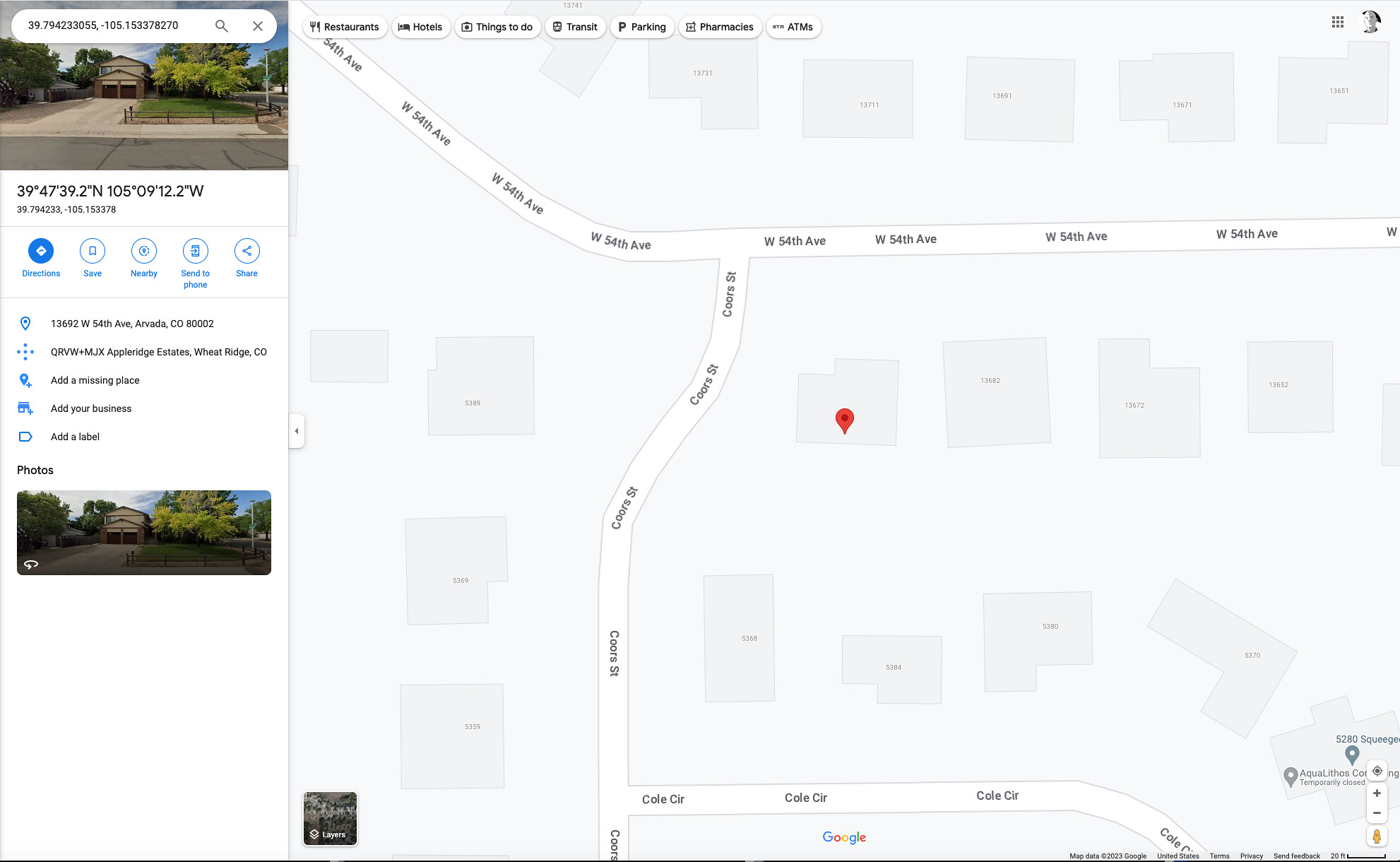This detailed image from Google Maps highlights a specific location with coordinates 39.794233055, -105.153378270. Displayed on the left side, the coordinate details are followed by an image of a house, surrounded by a sidewalk and road, located at 13692 West 54th Avenue, Arvada, Colorado, 80002, within the Apple Ridge Estates in Wheat Ridge, Colorado. The map interface also includes options like 'Directions,' 'Save,' 'Nearby,' 'Send to Phone,' and 'Share.' Additionally, there are prompts to 'Add a missing place,' 'Add your business,' and 'Add a label,' along with a street view photo of the house.

On the right side, the map in black and white shows West 54th Avenue beginning at the upper left-hand corner, extending downward about a fourth of the way, then turning and heading straight across the map. Connecting to West 54th Avenue is Coors Street, which runs down to the bottom of the screen. Cole Circle branches off Coors Street towards the bottom. The map details also include small numbered markers indicating various houses within the area.